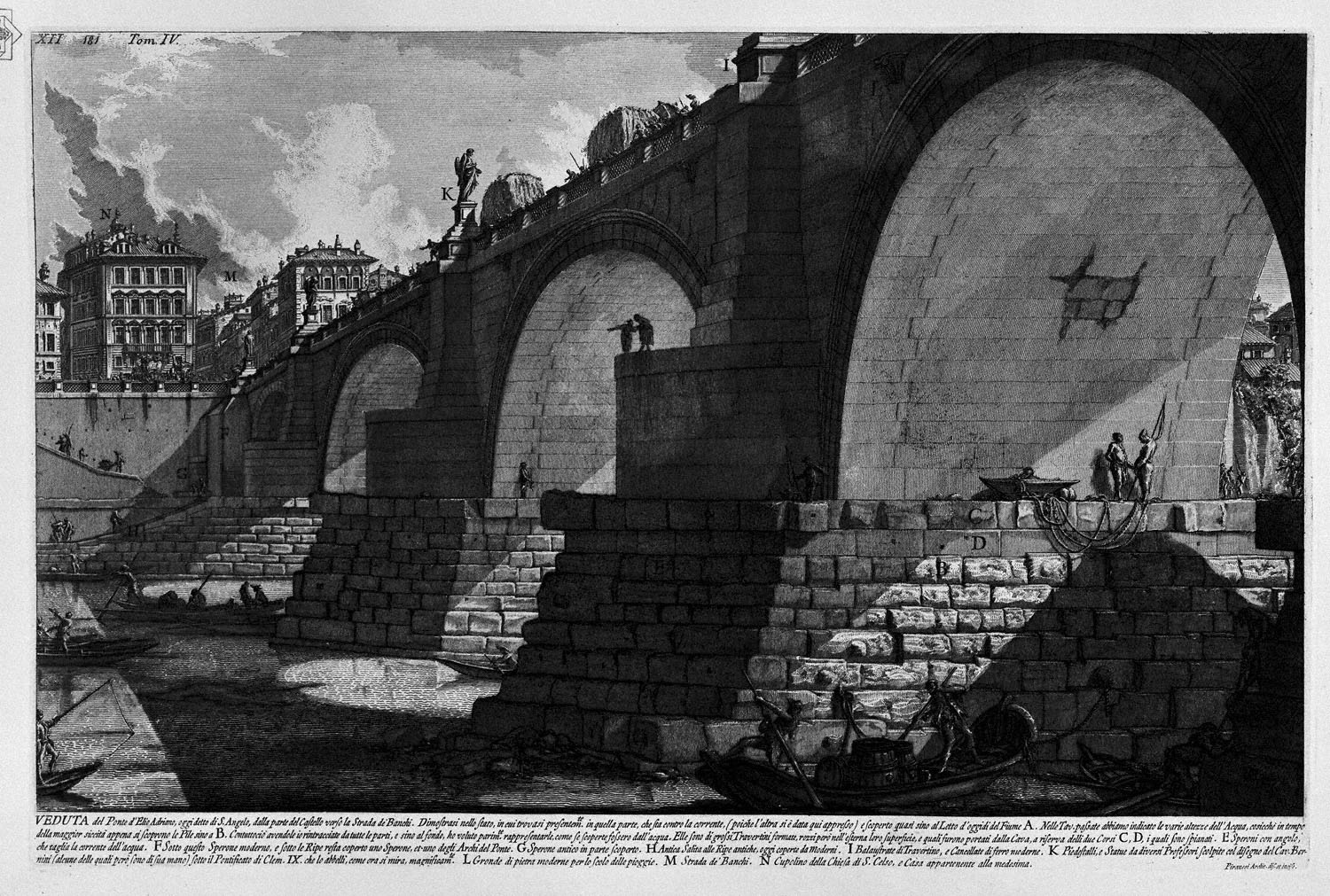The black and white pencil drawing-like illustration depicts a medium-length stone bridge with prominent thick buttresses. The composition places the first buttress on the right-hand side, where couple of people are barely visible sitting at its base. To the left, the bridge extends with two more stone buttresses leading towards the distance. The scene below the bridge includes several people in boats on the river. Above the structure, human figures and carriages are visible crossing the bridge, with city buildings rising in the background on the upper left side, under an open sky. The image, reminiscent of a textbook painting or print, has small, illegible text at the bottom, suggesting it might be an excerpt from a detailed textbook or historical document.